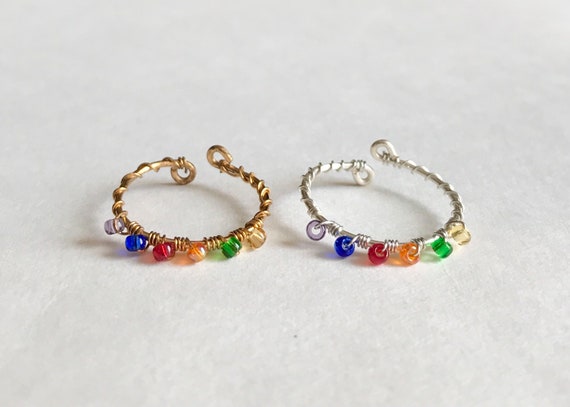This indoor color photograph captures two earrings displayed side-by-side on a stark white background, highlighting their intricate details. The earrings are made from thin wire, with one earring fashioned in gold and the other in silver. They are showcased in a three-quarter view, displaying their detailed design elements prominently. Each earring prominently features six colored beads arranged in an identical sequence: clear, blue, red, orange, green, and clear. This pattern is consistently replicated on both earrings. Encircling each loop is a delicate wire spiraled around its circumference, reinforcing the impression that these pieces are handcrafted. Despite their meticulous design, the earrings exude an aura of inexpensive, perhaps even homemade, jewelry, suggesting they are not of high quality. These adornments, with their vibrant beads and wire-wrapped design, might indeed be an amateur creation, possibly photographed for online advertisement against the simple white background.